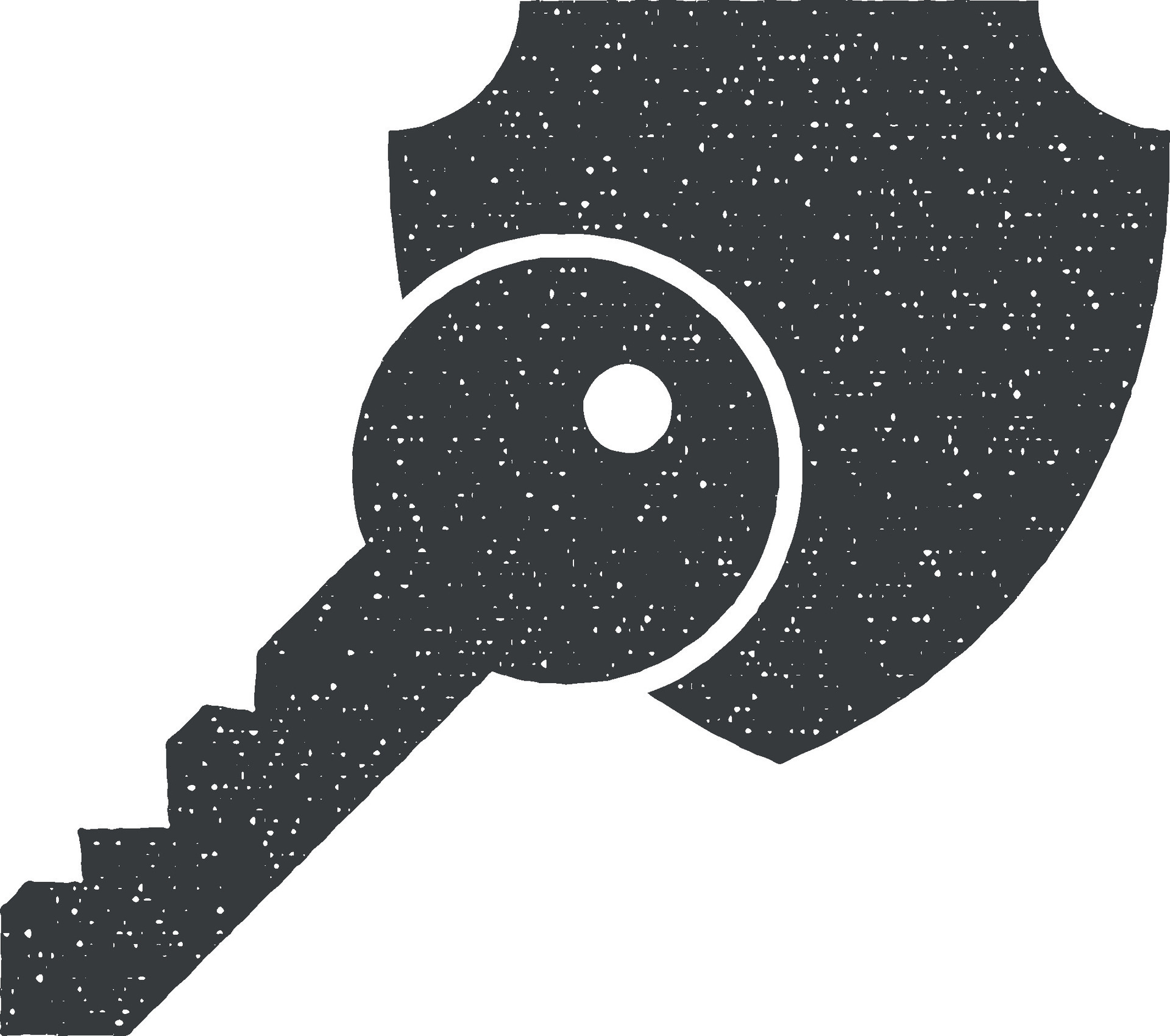The image is a graphic design featuring a dark gray key inlaid against a matching dark gray shield, set on a plain white background. The design elements include a key with four jagged teeth at the bottom edge and a round hole at the top, positioned such that the hole aligns with the middle of the shield. Both the key and the five-sided shield are adorned with randomly dispersed white dots that create a speckled pattern. The shield, with a straight top side and varying curved sides, features a concave semicircle cutout that conforms to the top rounded corner of the key. The shield covers a significant portion of the key, with the overall icon occupying approximately 80% of the image, leaving the remaining 20% as solid white space.